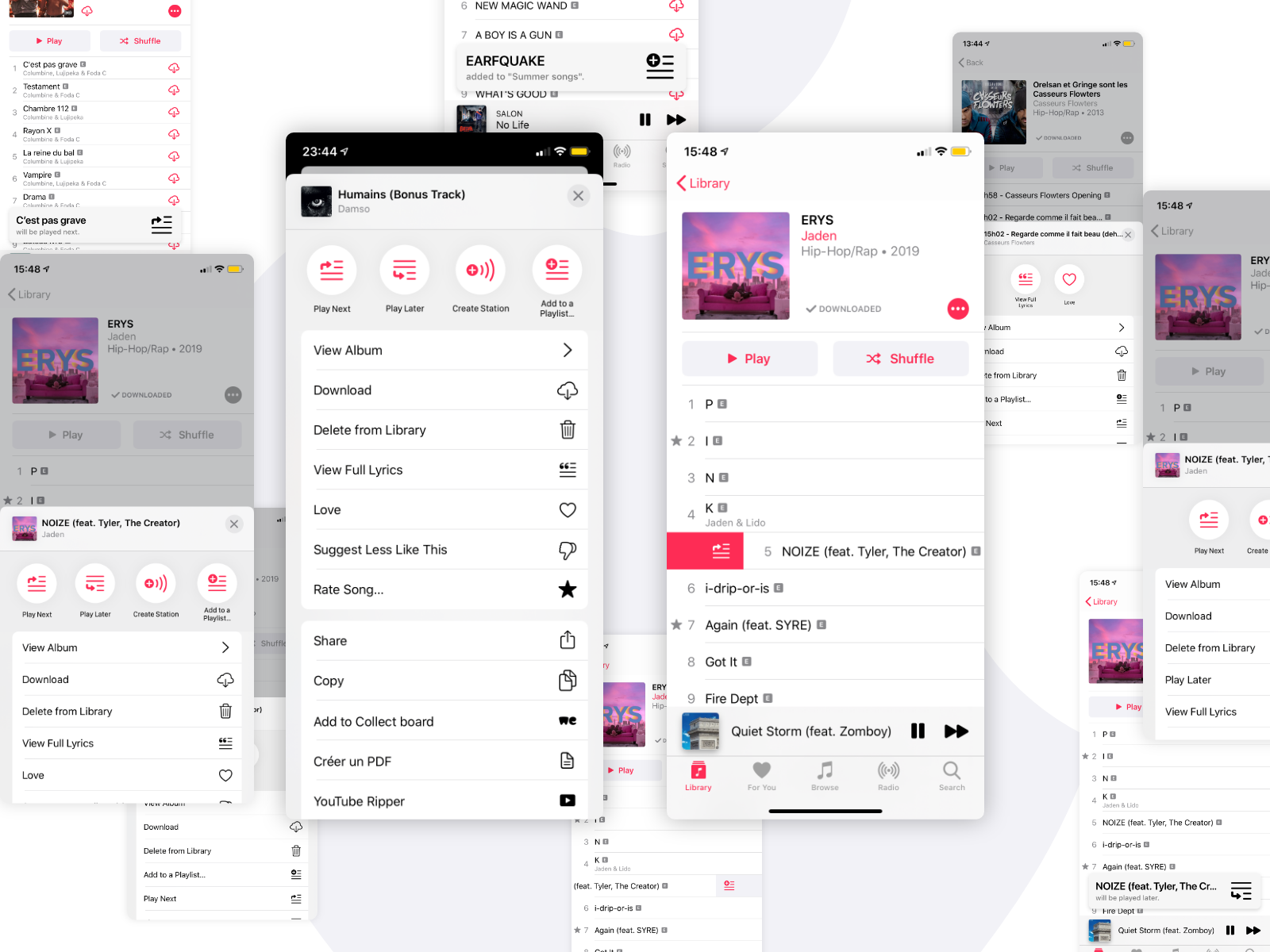A cluttered desktop screenshot reveals an array of overlapping mobile device windows. The central focus showcases two prominent windows: the one on the left displaying options such as "View Album," "Download," "Delete from Library," "Full Lyrics," "Love," "Suggest," and "Like" for a 'Bonus Track.' To its right, another window titled "E-R-Y-S, Jaden Hip Hop" is centered on the track "N-O-I-Z-E," offering play and shuffle functionalities. Overlaid in the background, additional windows hint at more music-related content, with titles like "new magic wand," "boy, is a gun," and "ear quake" visible. The overall impression is a busy, music-centric digital workspace on a mobile device.